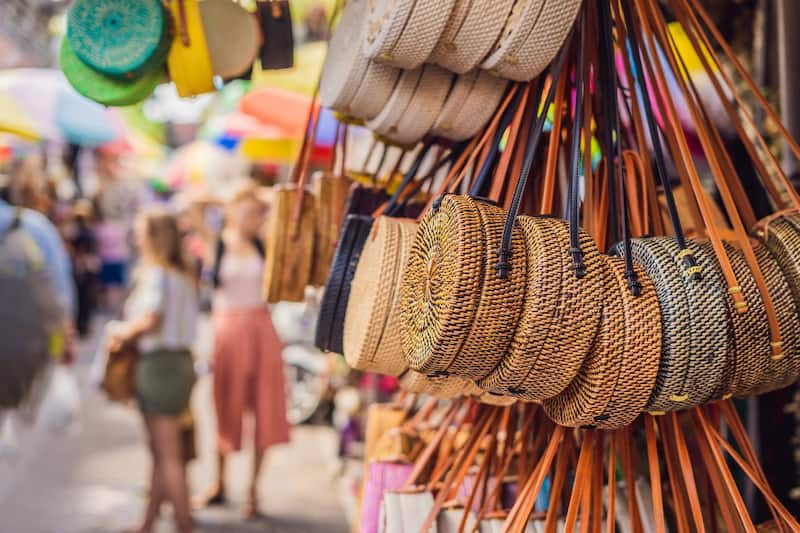This outdoor image depicts a bustling marketplace with a focus on circular, handwoven purses displayed prominently on the right-hand side. The intricately crafted purses, which appear to be made from thin reeds, feature tiny compartments and are adorned with long leather straps in shades of black and brown. The bags span a spectrum of colors, including red, white, black, green, blue, and various neutral tones like tan, beige, and browns. The top rows display purses in more muted hues, while more vibrant colors, such as pinks and greens, can be spotted on the lower rows. On the left-hand side, the background is blurred, revealing the indistinct forms of two women shopping and a mix of multicolored items that add to the lively atmosphere of the bazaar.